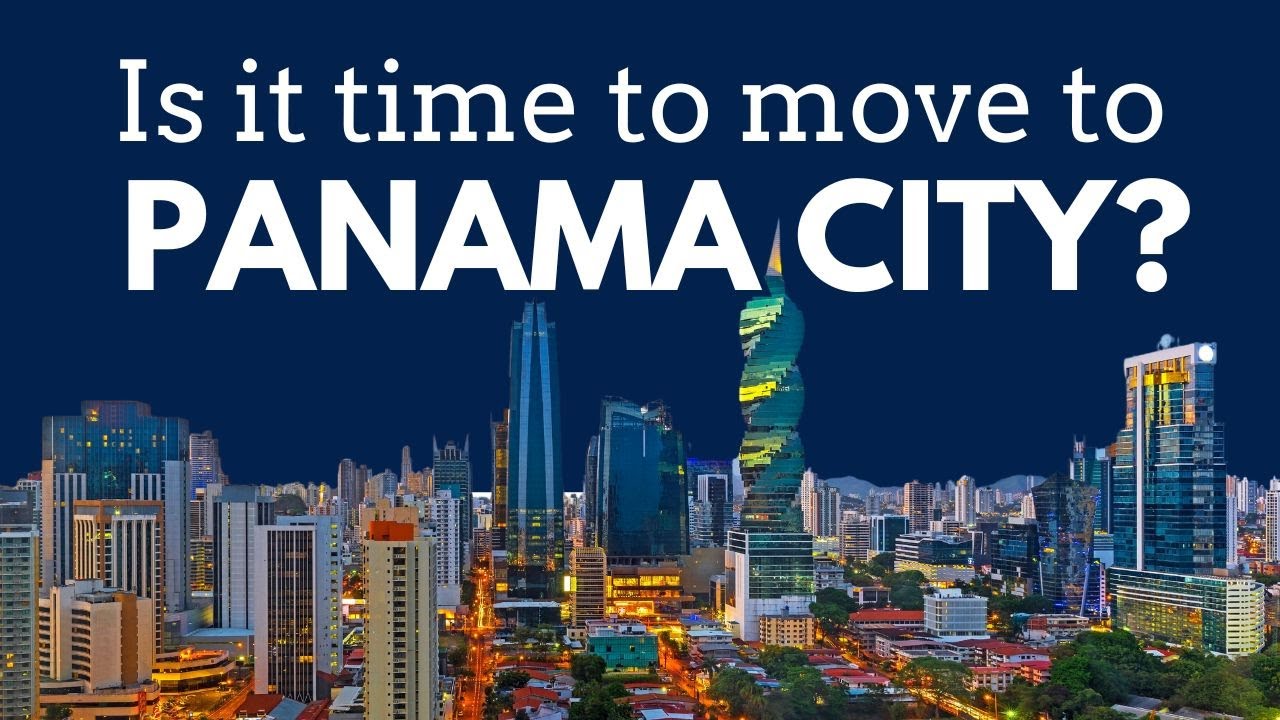A digitally-rendered image of Panama City's skyline dominates this scene, blending artistic elements with impressive architectural detail. The top portion of the image features a dark navy blue background that gradually transitions into the bustling cityscape below. Prominent in the foreground are four towering skyscrapers, with one unique structure at the center showcasing a distinctive twisting design as it ascends into the sky.

These colossal buildings, although taller, are complemented by numerous other high-rises that create a dense urban setting. One particularly striking skyscraper, with a pointed peak, dramatically divides the text "Panama City," which is superimposed in bold white letters. Above, the smaller and less prominent text reads, "Is it time to move to," leading into the larger, thicker font of "Panama City?" with a similarly bold question mark, all set against the building’s pointed architecture. The entire composition captures the modern allure of Panama City, inviting viewers to ponder the possibility of relocating to this vibrant metropolis.